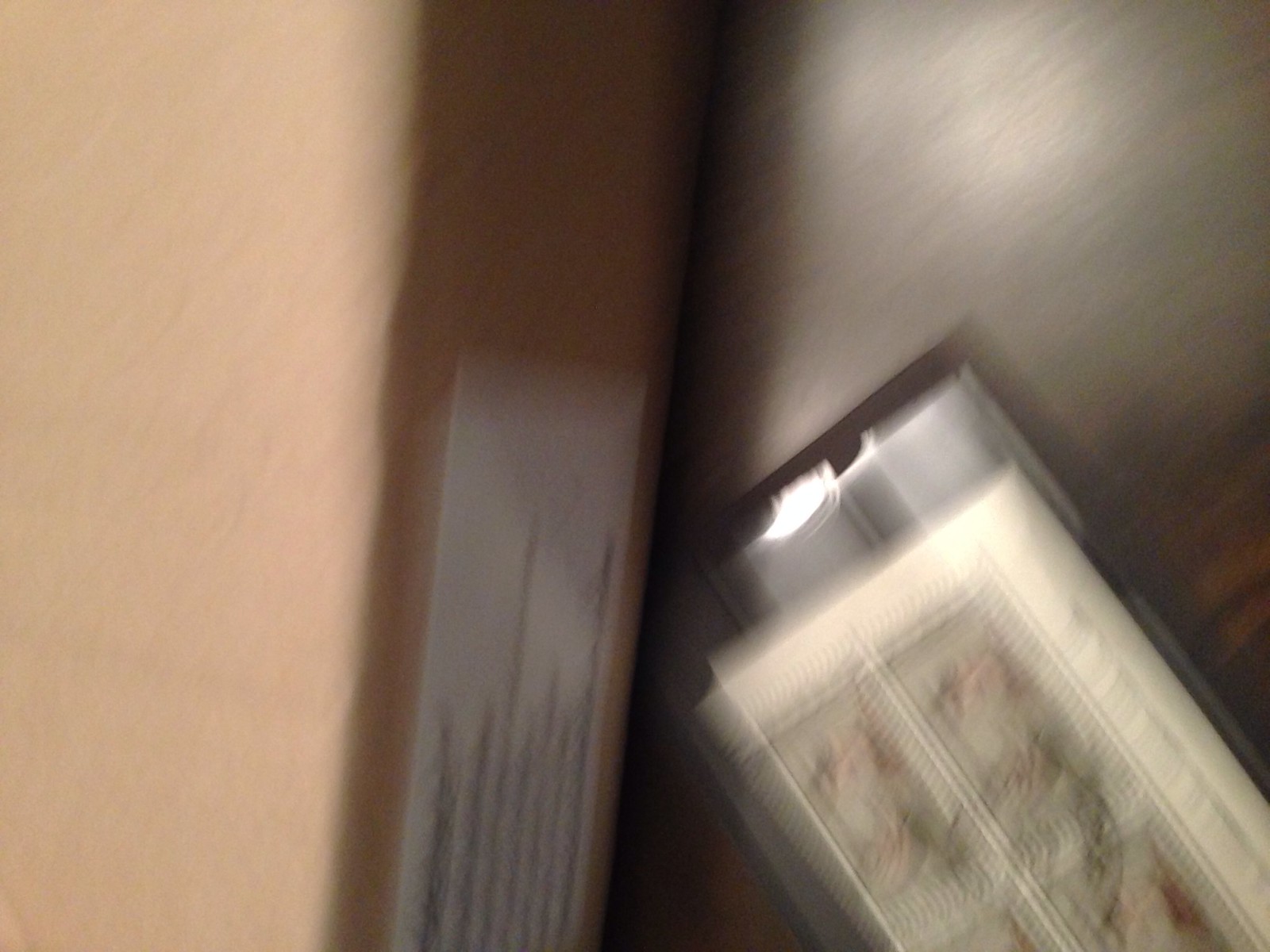This extremely blurry image appears to depict a scene with multiple layers and objects. On the left side, a tan or beige segment dominates, possibly hinting at the side of a box. There seems to be a sticker or label here with roughly seven lines of barely discernible text. Moving towards the center, a vertical brown strip emerges, potentially made of wood, embedded with a vertical silver metal placard. This part is darker with some light inexplicably shining down from above. To the right side of the image, a lighter section comes into view, where it appears to feature pieces of white paper with floral print, containing hints of pink and green leaves. These papers could be illustrations or part of a comic strip, potentially encased in a plastic package. Overall, the image suffers from significant motion blur, making precise details difficult to ascertain.